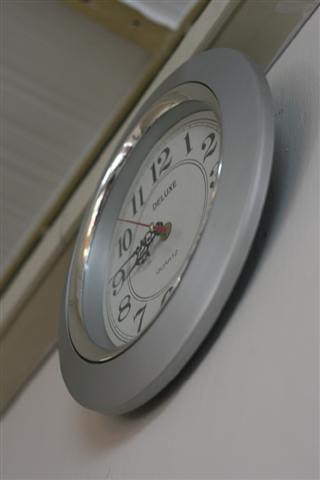Caption: 

A close-up view of a vintage circular quartz wall clock, prominently featuring the brand "Deluxe" on its face. The clock, with its unassuming yet classic design, showcases a silver-gray bezel with a chrome trim lining the inner edge, giving it a subtly aged appearance. The face of the clock is an off-white color, adorned with simple yet decorative numbers that enhance its nostalgic charm. The perspective of the photo suggests it is mounted high on a wall, likely above a blackboard or teaching area, in a room that appears to be commercial or educational in nature. The ceiling, visible above the clock, adds to the context of the setting, indicating a functional space used for learning or activities. The clock’s straightforward analog design contrasts with its timeless elegance, making it a practical yet aesthetically pleasing fixture on the wall.